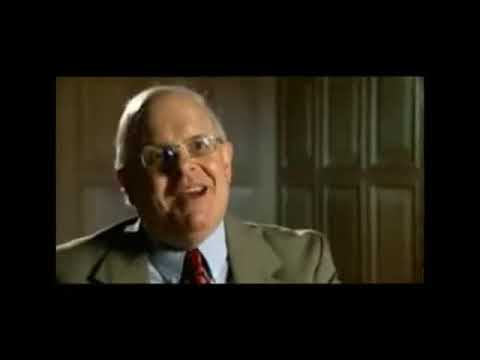The image depicts an older man with a receding hairline and white comb-over hair, wearing small rectangular glasses that reflect the light. His clean-shaven face shows a slight smile, revealing his upper teeth as he appears to be talking. He is dressed in a light gray or tan suit over a light blue collared shirt, paired with a red tie. Positioned in front of a panelled yellow wall, which possibly features closet doors with square designs, the scene is framed by a solid black border. The lighting creates a subtle shadow on the left side of his face, while his forehead and right cheek catch the light, adding depth to his expression.